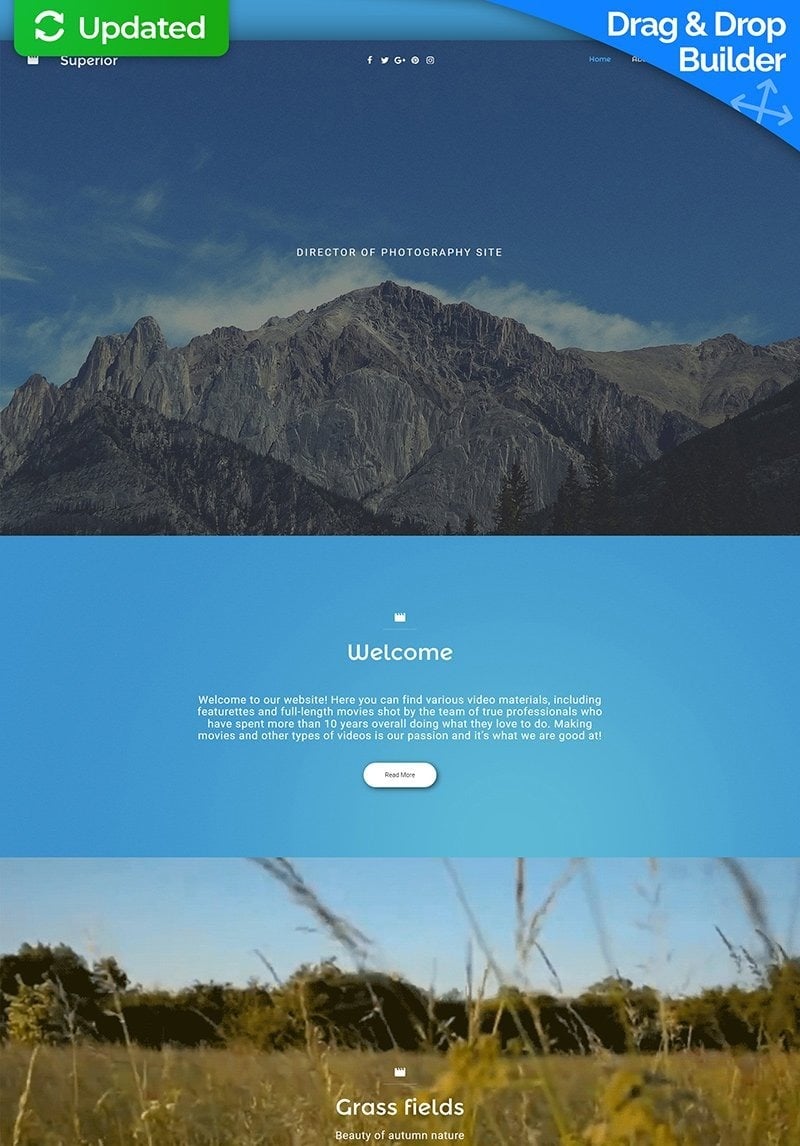This image portrays a template for a website builder, specifically designed for a Director of Photography website. In the top right corner, a small triangular cutout is labeled "Drag and Drop Builder," indicating the customizable nature of the design.

Central to the layout is a prominent title, alongside a secondary title that reads "Director of Photography Site." Below this, a welcoming message greets visitors: "Welcome to our website. Here, you can find various video materials, including featurettes and full-length movies shot by a team of true professionals who have spent more than 10 years doing what they love. Making movies and other types of videos is our passion, and it's what we're good at." An option to "Read More" is provided immediately following this message.

The layout is visually divided into two sections featuring large images. The upper section showcases a stunning mountain range under a sky with scattered white clouds. The lower section displays serene grass fields bordered by green trees, with a clear blue sky in the background. At the very bottom of the page, the text "Grass Fields: Beauty of Autumn Nature" further describes this image.

Overall, this template serves as a detailed example of how the website could look, emphasizing both visual appeal and informative content for a photography-focused site.